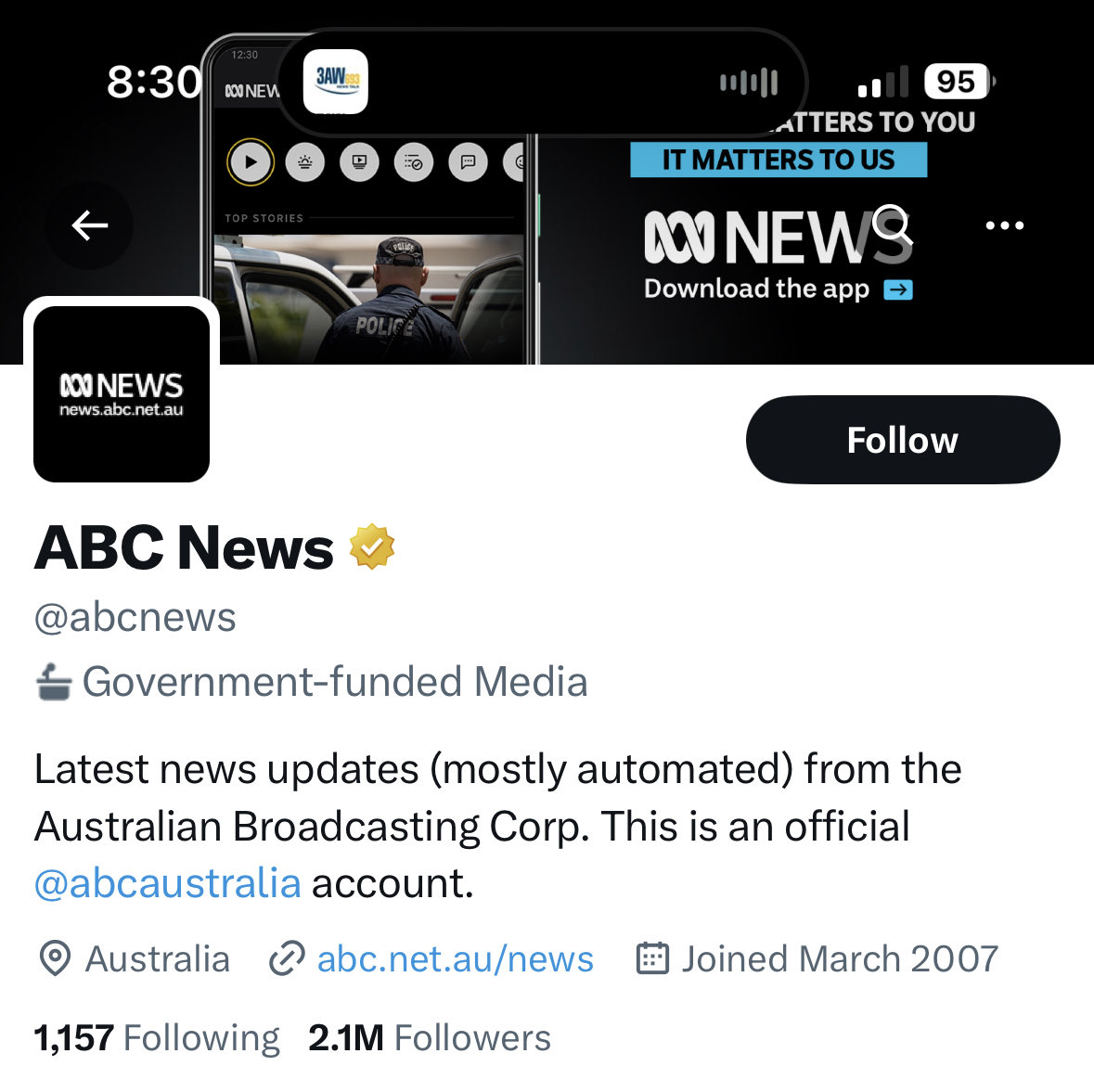This image is a screen capture of what appears to be the ABC News Twitter page. At the top right corner, the time is displayed as 8:30, alongside a battery indicator showing 95% and three white dots representing network connectivity. An arrow pointing backward suggests navigation options.

The header features a black banner with an advertisement showcasing a simulated smartphone screen filled with gray circles. A police officer is pictured with his back to the camera. White text on the banner reads, "If it matters to you," followed by black and blue text that reads, "it matters to us." Beneath this, the banner encourages users to "Download the app," with a blue and gray downward arrow accompanying the suggestion. Next to the word "News" is a symbol resembling an infinity sign.

Below the header, a rectangular black box with white text contains the infinity symbol again, the word "News," and the URL "news.abc.net.au." To the right, a black and white "Follow" button is prominently displayed.

Further down, the account's profile information is detailed. A gold check mark appears next to "ABC News" with the handle "@ABCNews." A podium icon follows, indicating the account as "Government Funded Media." Additional information states, "Latest News Updates, Mostly Automated, from the Australian Broadcasting Group." The bio confirms this as an official account of ABC Australia, and a location pin points to Australia. A pay-per-click icon is followed by the website link "abc.net.au/news," and a calendar icon notes that the account joined in March 2007.

The stats at the bottom reveal that the account is following 1,157 other profiles and has amassed 2.1 million followers.